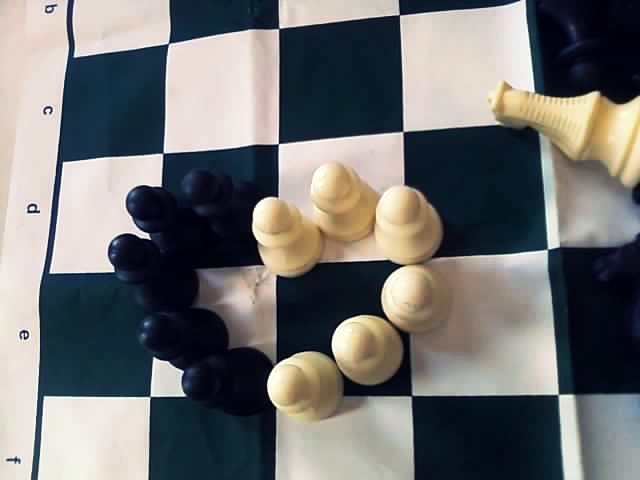The image showcases a cloth chessboard with a black and white checkered pattern, designed for foldability. Along the left-hand side of the board are columns labeled B, C, D, E, and F. At the center of the board, arranged slightly toward the bottom left, black and white pawns have been meticulously positioned to form a heart shape, with black pawns composing the left half and white (ivory) pawns the right half. On the far right side of the board, larger game pieces, which appear to possibly be a horse (knight) or king, and possibly another piece such as a rook or queen, are lying flat. The board itself sits on a surface that reveals a small, light gray triangular section in the upper left-hand corner of the image.